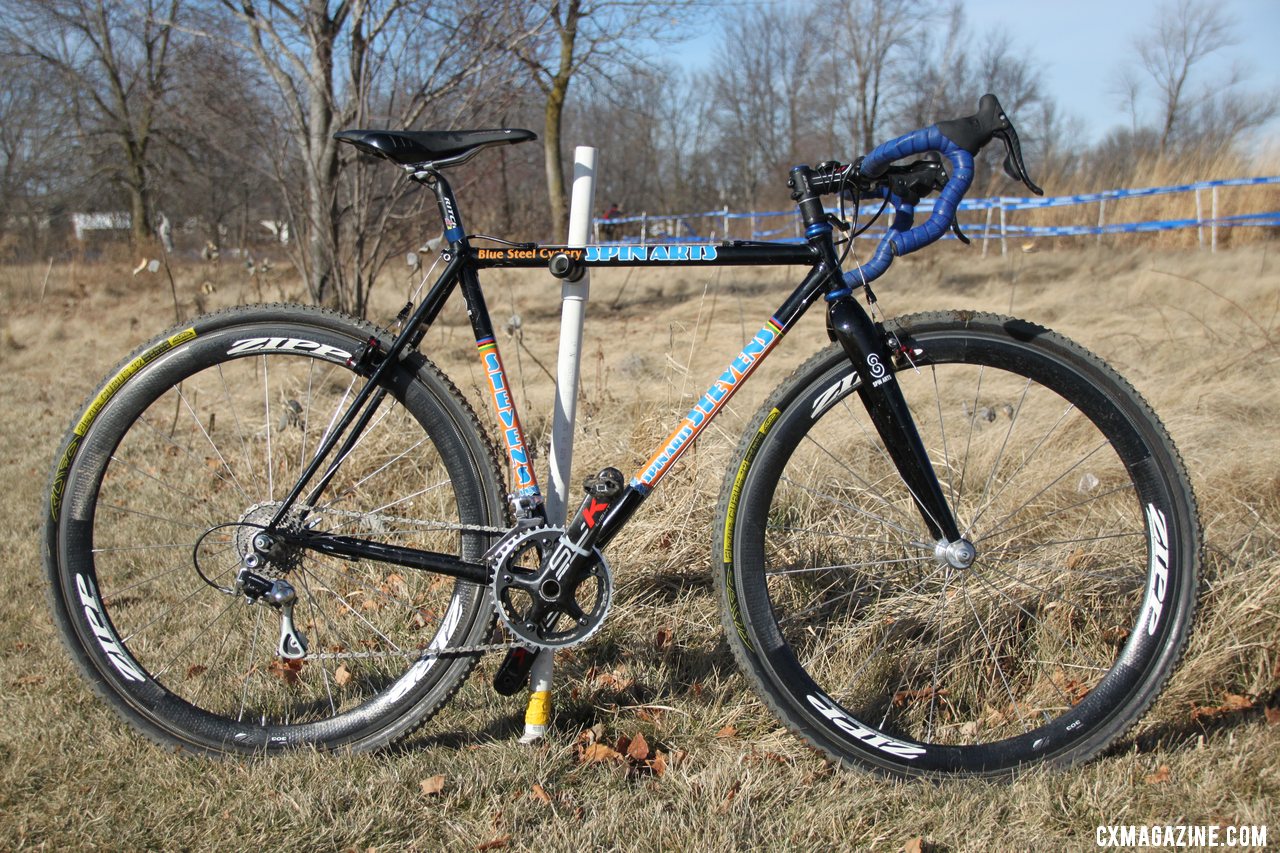This image showcases a close-up of a ten-speed road bicycle with a black steel frame adorned with various colorful sponsor decals. Notable markings include "Spin Arts" and "Blue Steel Cyclery" in blue and gold lettering on the top tube and "Stevens" in blue on a yellow background near the gearbox and crankshaft area. The bike features blue handlebar tape on traditional drop-style road handlebars, black brake levers, and a black saddle seat. The wheels are fitted with ZIPP tires, indicated by the white ZIPP lettering on the tire sides. The bike is propped up against a white tubular post situated in a meadow of brownish, straw-like grass. The background features barren trees and a blue wooden fence with white posts, providing a wintry atmosphere. The corner of the image includes the watermark "CXMagazine.com."